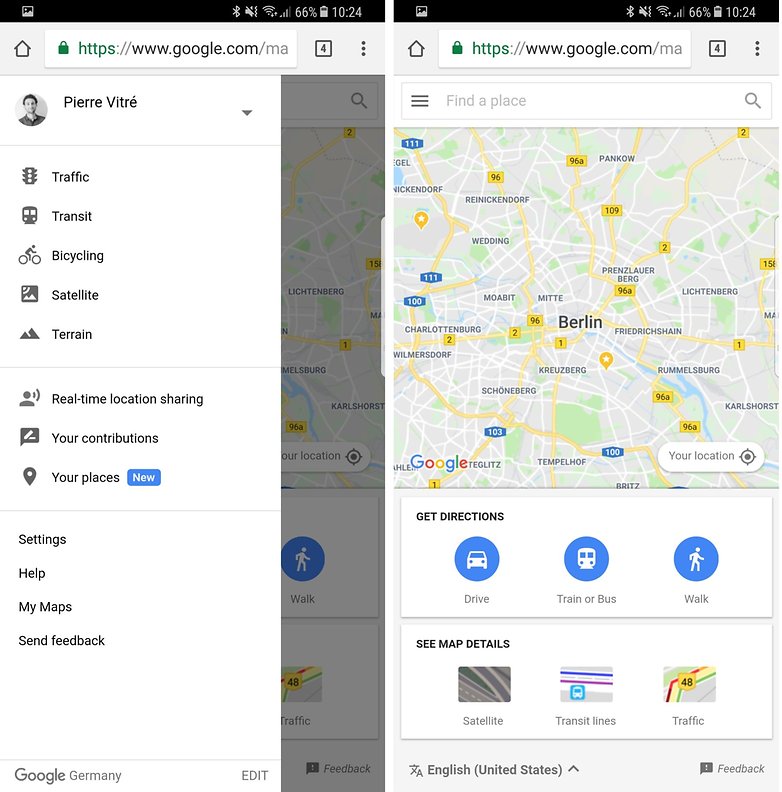The image features two mobile screenshots of a Google Maps interface.

On the left side, the screenshot shows the expanded left panel. At the top, it displays the username, followed by a list of options such as Traffic, Transit, Bicycling, Satellite, and Terrain. Below these options, there are additional features like Real-time Location Sharing, Your Conditions, Your Places, Settings, Help, My Maps, and Send Feedback. At the bottom of this panel, the text "Google Germany" is visible to the left, with the word "EDIT" in capital gray letters to the right.

On the right side, the screenshot presents the main map view focused on Berlin. This large map occupies the majority of the screen, with the Google logo situated at the bottom left corner and a white bubble labeled "Your location" in the bottom right corner. Beneath the map are two white boxes. The top box features the "Get directions" option along with three icons representing different modes of transportation: Drive, Transit (train or bus), and Walk. The second box, positioned at the bottom, displays the "See map details" option with three corresponding thumbnails for Satellite, Transit times, and Traffic.